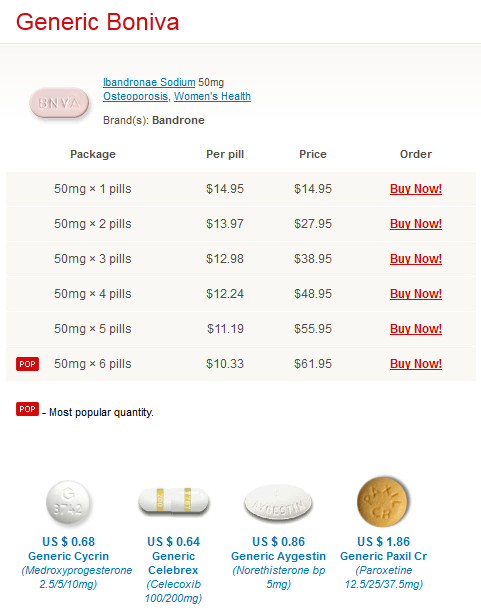The image features an advertisement for generic Boniva, a prescription medication. The top of the advertisement prominently displays "Generic Boniva" in red text. Below that, there is a box showcasing an image of the pill, which is pink and engraved with "VA". The medication is labeled as "Ibandronate Sodium, 50 mg," and is intended for women's health, specifically for the treatment of osteoporosis.  

The brand name "Bandrone" is mentioned, with "Sodium" and "Osteoporosis Women's Health" each provided as clickable hyperlinks. Below the description, the advertisement is organized into four columns: "One Per Package," "One Per Pill," "Price," and "Order."

The pricing structure is detailed as follows:
- One pill costs $14.95.
- Two pills cost $13.97 each, totaling $27.95.
- Three pills are priced at $12.98 each, totaling $38.95.
- Four pills cost $12.24 each, totaling $48.95.
- Five pills are priced at $11.19 each, totaling $55.95.
- Six pills, marked as the "Most Popular Quantity," are $10.33 each, totaling $61.95.

Underneath the main product details, there is a legend in red text indicating "POV" as the most popular quantity.

Additionally, the advertisement includes images and prices for four other generic medications:
- Generic "Cicerin" for $68.
- Generic "Celebix" for $64.
- Generic "iGestin" for $86.
- Generic "Paxil" for $1.86.

Each of these medicines appears with its price, offering consumers a comparison to make informed purchasing decisions.